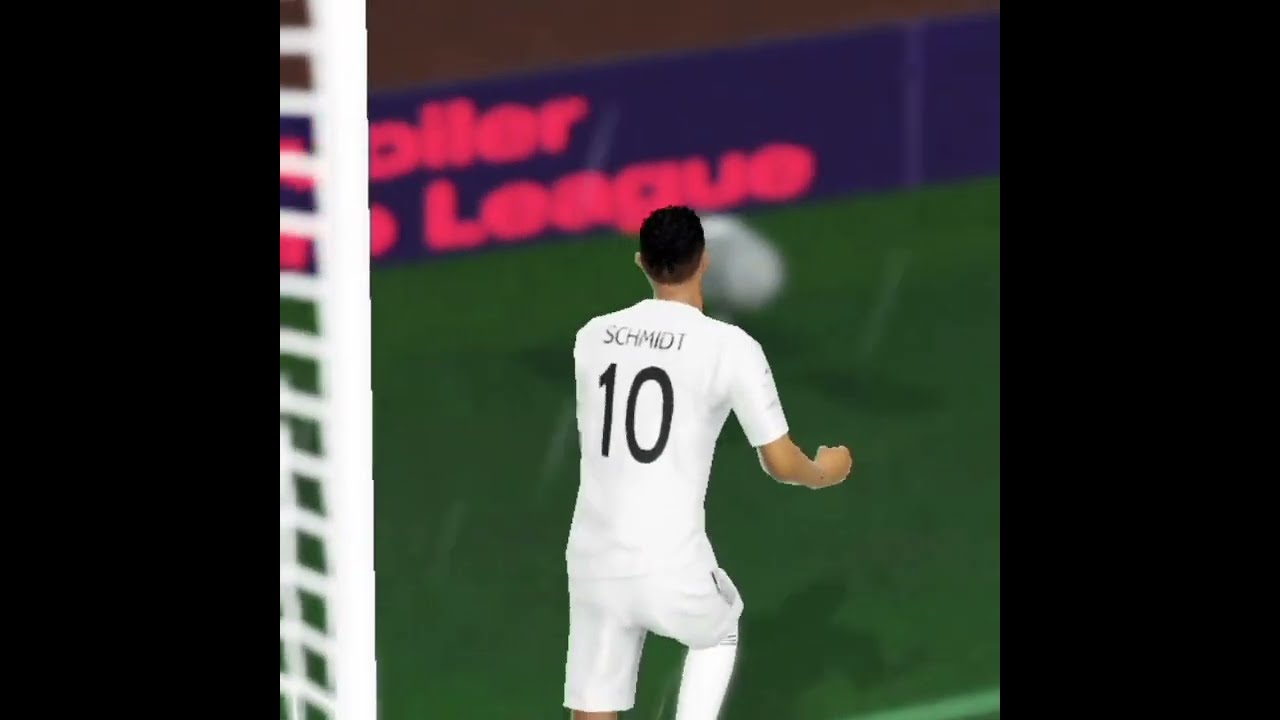In this detailed image, we see the back view of a soccer player, identified as Schmidt, wearing the number 10 on his white jersey. He has short black hair, and his last name, SCHMIDT, is printed in black above the number on the jersey. The scene takes place on a green soccer field with a white ball near him. A blurry goalpost and white netting are slightly visible on the left side. A notable feature in the background is a horizontal blue banner with partially visible red text that reads "OLLER" and "League" in pink letters. The image is framed by thick black vertical bands on each side, suggesting that it might be a screen capture from a video game.